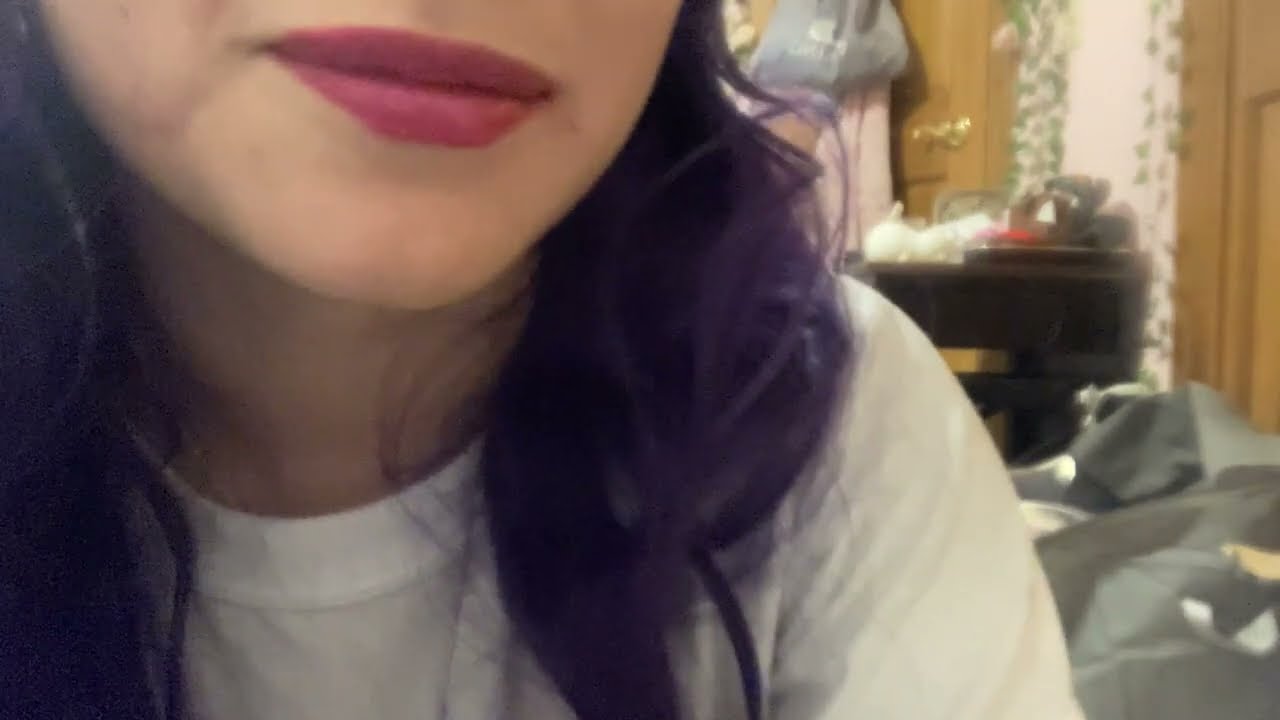In this indoor photograph, a close-up of a woman's lower face and upper chest dominates the left side. She is wearing black lipstick and a white crew neck T-shirt, with her long, wavy black hair cascading down. Only her mouth and the area just below her shoulders are visible. The setting is detailed with two brown wooden doors on the right side, one near the center adorned with a plastic bag and some plain clothes. Between the doors is a black shelf or table, while the floor in front of the door on the right is occupied by a gray blanket. The walls are white, adding to the room's simplicity.